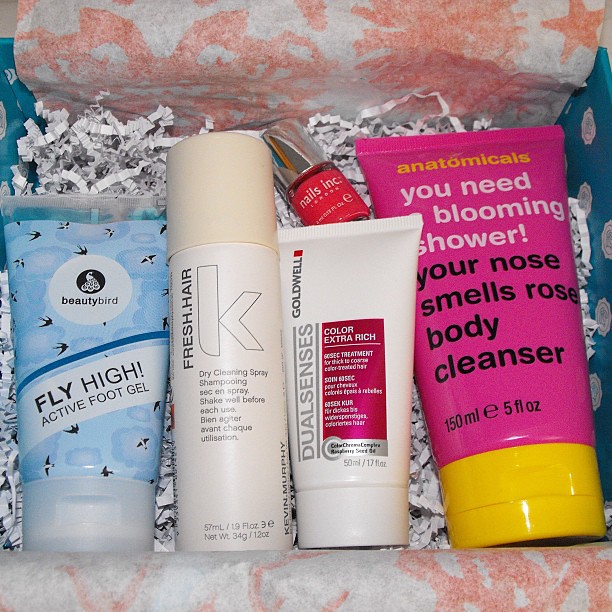This image showcases an unboxing moment of a small blue cosmetics gift box, perfect for an Instagram post. The interior is lined with shredded white paper for cushioning and decorated with pink and white splotched tissue paper. Several beauty products are neatly arranged inside.

On the far left, there is a blue tube labeled "Beauty Bird" within a white circle, with the text "Fly High Active Foot Gel" and a white cap. Next to it, a cylindrical beige container displays the brand name "Kevin Murphy" and "Fresh Hair Dry Cleaning Spray Shampoo." Further to the right is a white tube labeled "Goldwell" along with "Dual Senses Color Extra Rich Treatment," featuring a pinkish bar and a white cap. Above this, there's a small bottle of red nail polish with a silver cap.

To the far right lies the largest item, a pink tube with a yellow cap labeled "Anatomicals." The tube's text reads "You Need a Blooming Shower" in white letters and "Your Nose Smells Rose Body Cleanser" in black, detailing its 150 ml volume. Each product adds to the diverse selection of beauty items, presented thoughtfully within the charming gift box.